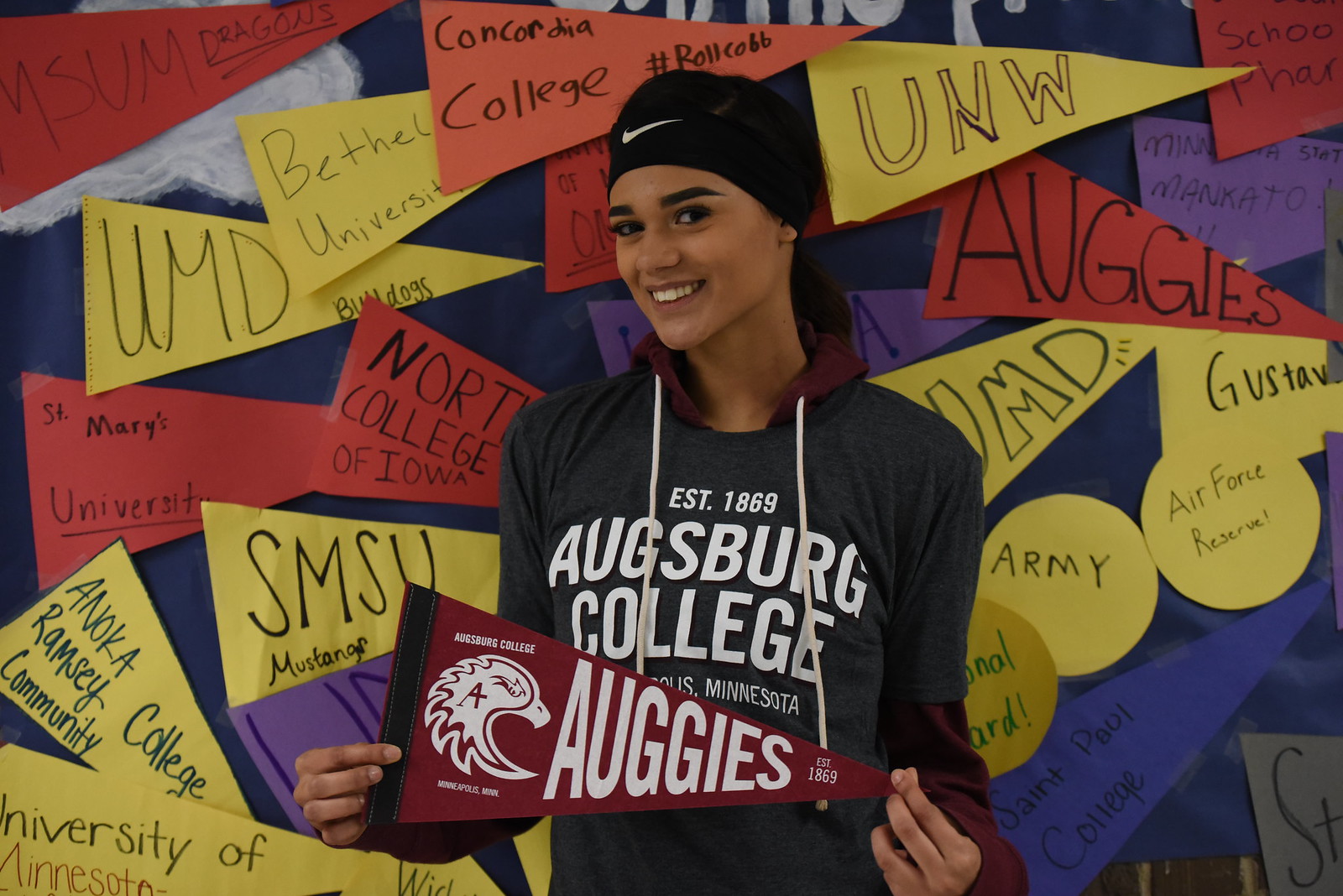The image features a young woman with dark hair and eyebrows, smiling as she stands in the middle of the photograph. She is wearing a layered outfit that includes a maroon long-sleeve hooded sweater with white drawstrings, over which she has a gray t-shirt that reads "Established 1869 Augsburg College, Minnesota." On her head, she has a black Nike headband bearing a white checkmark logo. In her hands, she holds a maroon, white, and black pennant that reads "Augies Augsburg College" with an eagle logo and an 'A' at its center. The background is a blue wall decorated with numerous colorful pennants in red, yellow, blue, and other hues. These pennants display names of various institutions and organizations, including MSUM Dragons, UMD Bulldogs, Bethel University, St. Mary's University, Anoka-Ramsey Community College, SMSU, North College of Iowa, Concordia College, UNW, Army, Air Force Reserve, University of Minnesota, and St. Paul College. The overall scene suggests a celebratory atmosphere, possibly representing collegiate pride or an alumni event.